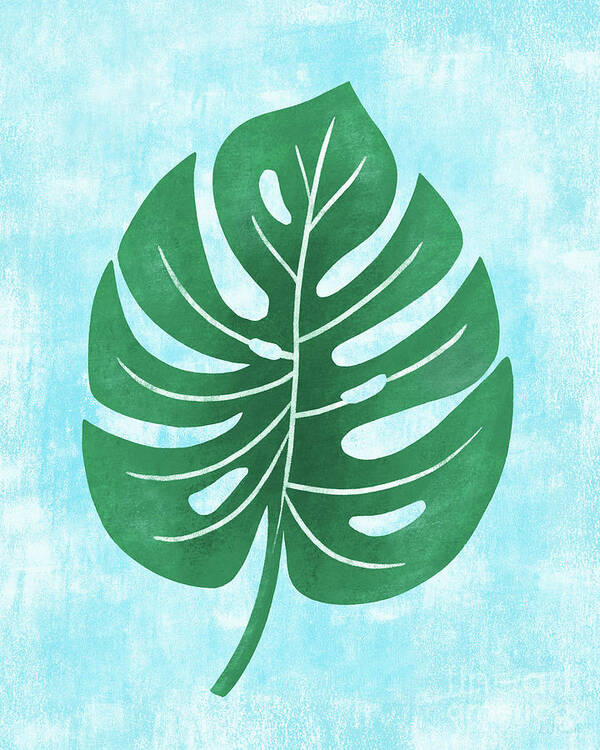The image is a detailed hand-drawn depiction of a large green leaf against a sky blue background with white cloud-like streaks. The leaf features a gradient of green, transitioning from a darker shade at the center to a lighter green at the edges. The central part of the leaf is almost black, emphasizing the gradient effect. The long green stem at the bottom leads up to multiple sections of the leaf, each showing intricate white lines representing the veins. The leaf also contains several holes, through which the sky blue and white background is visible, adding depth and realism to the drawing. The bottom right corner of the image includes some artistic text, indicating the origin or inspiration of the artwork.